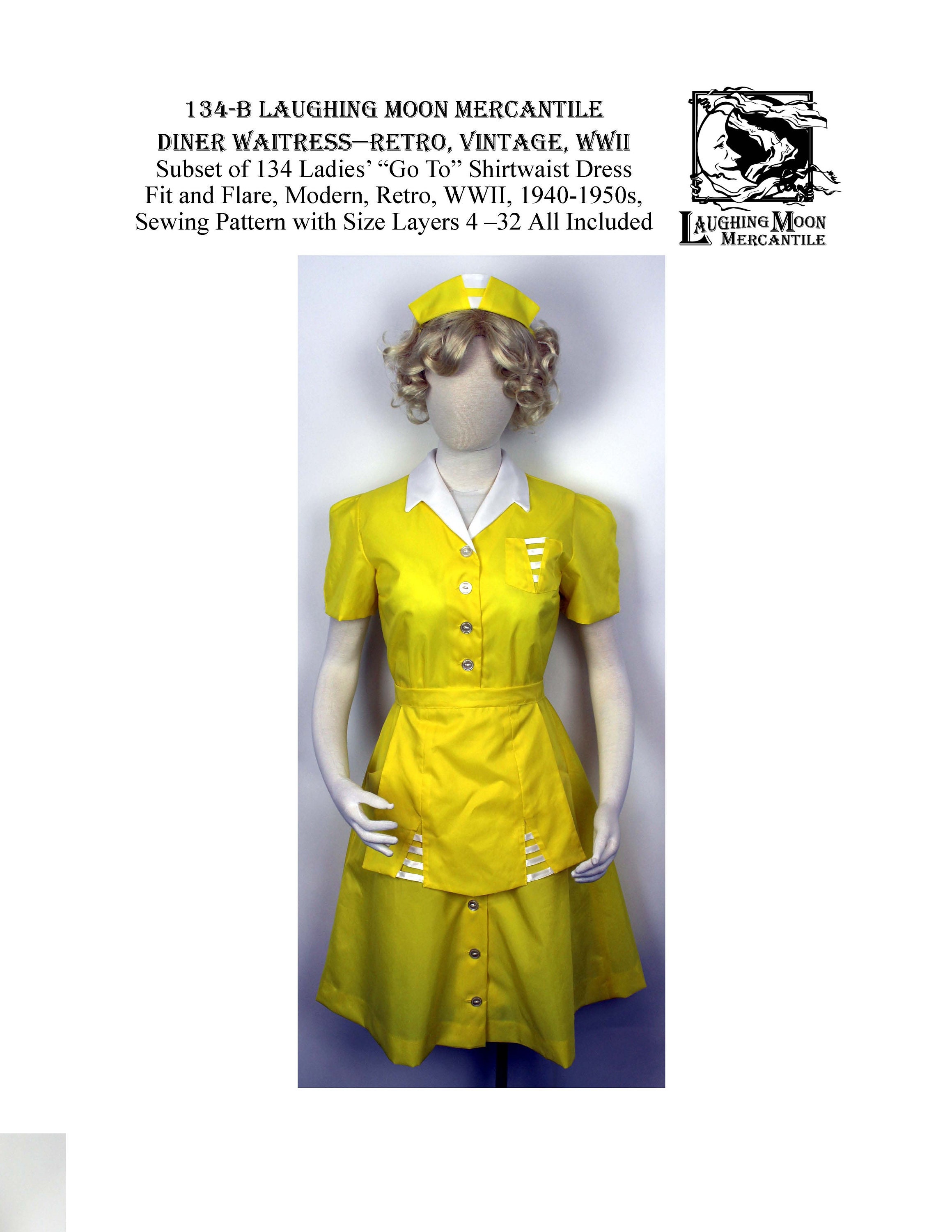The photograph showcases a central mannequin adorned with a bright yellow shirtwaist dress reminiscent of a retro, vintage 1940s-1950s diner waitress uniform. The mannequin sports a blonde, curly wig and is positioned on a stand without visible legs. The dress features short sleeves, a white collar, and white accents, including a modest apron and a pocket on the upper half. It buttons down the front and extends below the knees. Complementing the outfit is a small yellow waitress hat with white details. Above the mannequin, the text reads "134B Laughing Moon Mercantile, Diner Waitress, Retro Vintage, World War II, WWII, subset of 134, Ladies Go To, Shirtwaist Dress, Fit and Flare, Modern Retro, World War II, 1940s to 1950s, Sewing Pattern with Size Layers, 4-32, all included." To the right of this text sits the Laughing Moon Mercantile logo, depicting a smiling crescent moon. The background of the image is a simple white with some blue elements.